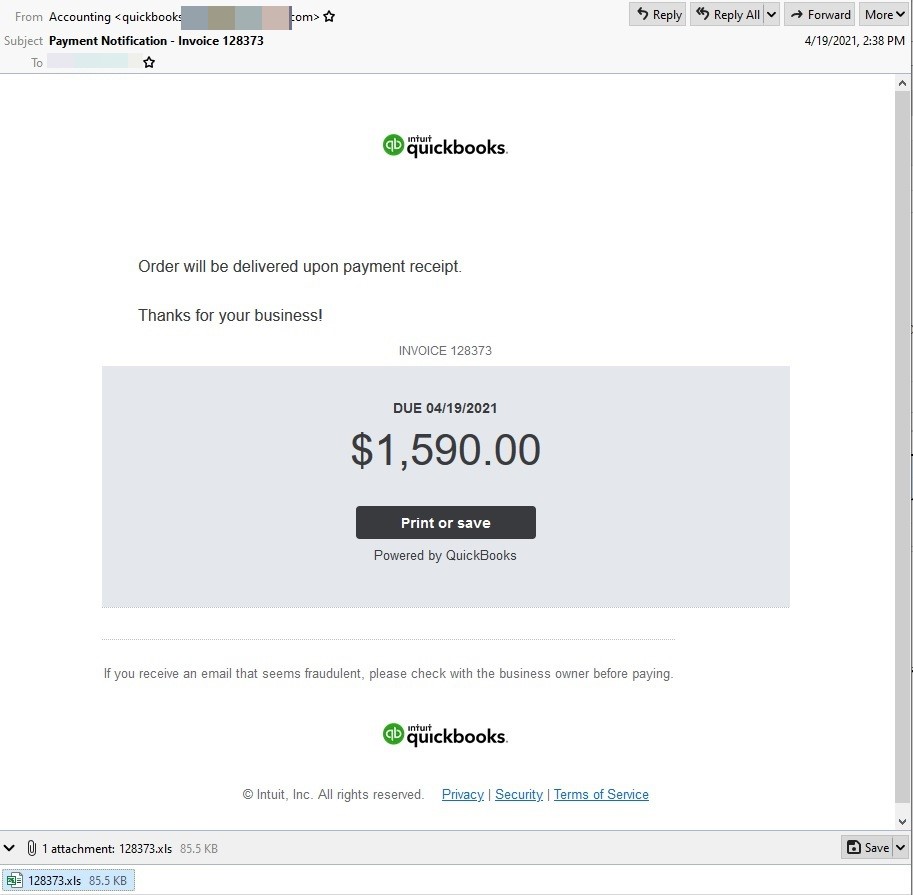The image depicts an email notification from Intuit QuickBooks. 

**Email Header:**
- **Upper Left Corner:** Features the Intuit QuickBooks logo. Part of the URL is obscured, displaying "...com."
- **Next Line:** Subject line reads "Payment Notification - Invoice 128373", with the number "2" partially obscured.

**Email Options:**
- **Upper Right Corner:** Contains buttons for "Reply," "Reply All," "Forward," and "More." The email timestamp is "4-19-2021, 2:38 PM."

**Email Body:**
- **Central Section:**
  - Prominent QuickBooks branding.
  - Text: "Order will be delivered upon payment receipt. Thank you for your business."
  - Details: "Invoice 128373, Due 4-19-2021, $1590."
  - Action Button: A black button with white font labeled "Print or Save."
  - Footer: "Powered by QuickBooks."

**Additional Information:**
- **Fraud Warning:** "If you receive an email that seems fraudulent, please check with the business owner before paying."
- **Copyright and Legal Information:** "Intuit QuickBooks", "Intuit Incorporated, all rights reserved," followed by links or references to "Privacy," "Security," and "Terms and Service."

**Attachment Section:**
- **Right Side Button:** A button labeled "Save."
- **Left Bottom Corner:** Shows a paperclip icon symbolizing one attachment named "128373.xls" with a file size of "85.5 KB."

This cleaned-up caption delivers a concise and thorough description of the email content, layout, and key details.